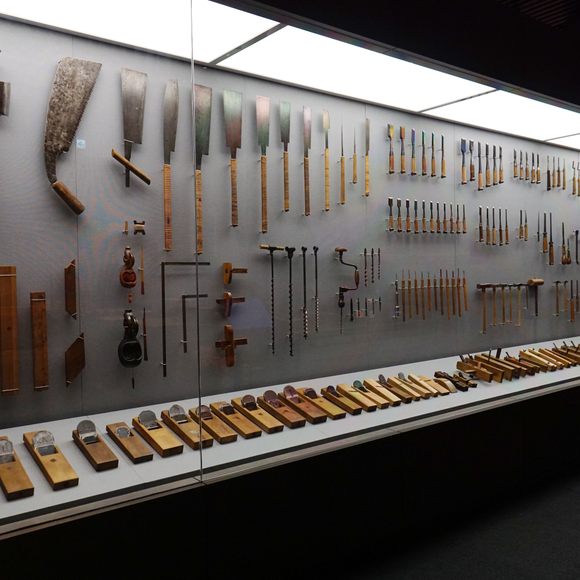This photograph captures a detailed and impressive display of wooden and metal hand tools, likely housed in a museum. The tools are carefully arranged in a large, glass-enclosed case that spans the entire image. Fluorescent lighting installed above the display highlights around a dozen different types of hand tools mounted on a medium gray (dove gray) wall. The tools, featuring long tan wooden handles and some silver metal ends, include various saws with trapezoidal and curved handles, hand drills, scrapers, picks, chisels, hammers, and different types of drill bits.

At the bottom of the case, on a black shelf, are several wooden blocks, possibly wooden planes, arranged side-by-side. Some of these blocks have holes or square cutouts, and a few feature metal parts. The array of tools, all meticulously organized, provides a fascinating glimpse into traditional craftsmanship and tool usage, all protected and showcased within the confines of the glass case.